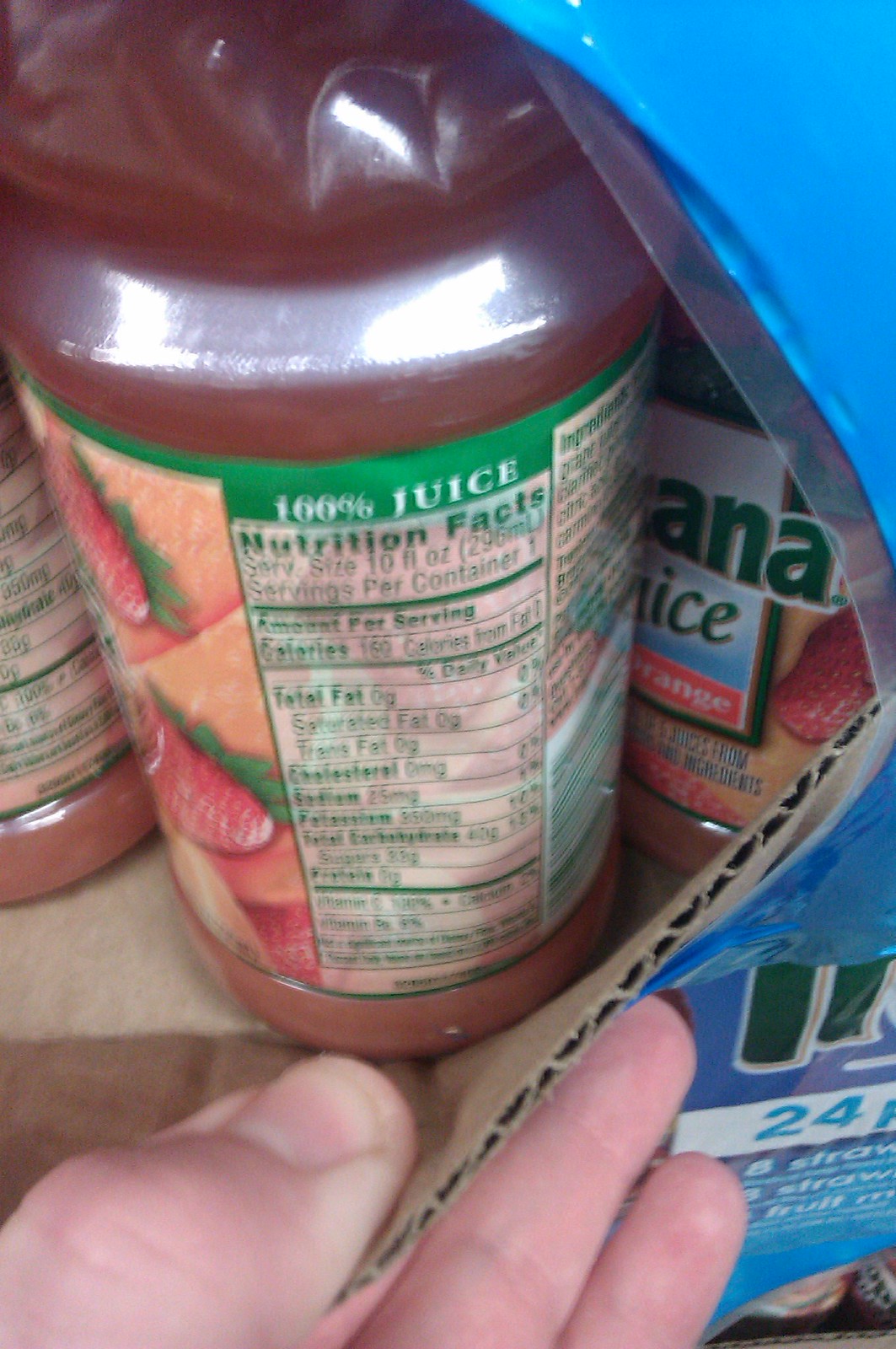In this close-up photograph taken in a store, we see a hand, most likely a man's hand with white skin, pulling back the cardboard and plastic covering of a case of drinks. The hand is revealing several plastic bottles of juice, particularly focusing on a bottle of Tropicana strawberry orange juice. The label on the bottle prominently displays images of strawberries and oranges, alongside the text "100% juice". Additionally, the image showcases the nutrition facts section of the bottle in detail. The information includes a serving size of 10 fluid ounces, with 160 calories, 0 grams of fat, 0 grams of saturated and trans fats, 0 milligrams of cholesterol, 25 milligrams of sodium, potassium content, 0 grams of carbohydrates, listed protein, and sugars.